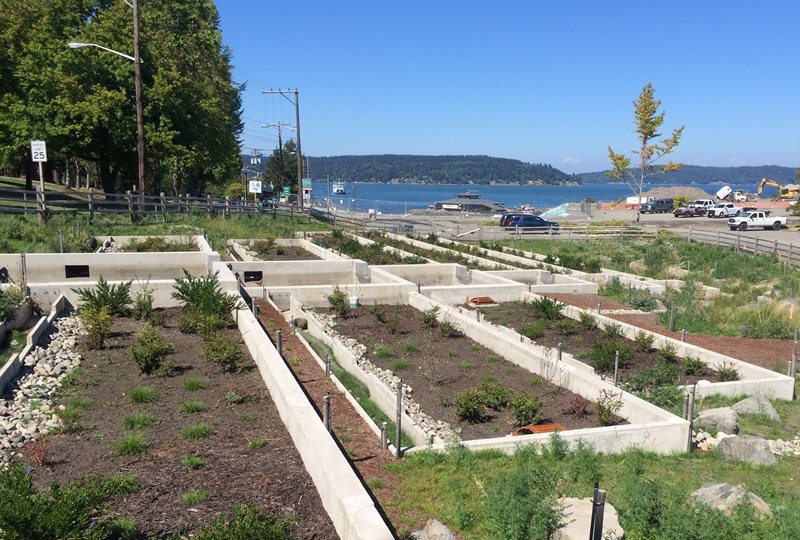This detailed photograph captures a tranquil coastal garden scene. In the foreground, there are rectangular white concrete garden beds filled with dark brown soil with small green tufts, suggesting early stages of plant growth. The ground surrounding the garden features patches of green and light brown. On the left side in the distance, a tall copse of green trees stands in front of a wooden fence, next to a white rectangular speed limit sign indicating 25 miles per hour. A road extends from the right, diminishing into the center of the image, with several vehicles including a white pickup truck, a blue sedan, and a few other cars. To the center right, a tree with reddish-green leaves stands prominently. Nearby, a bright yellow backhoe operates in the far right corner along with several white trucks. At the shore of a serene blue body of water, a hexagonal building with a gray roof is observed. In the water itself, a small white ship is approaching the viewer. Beyond the water lies a tree-covered hilly strip of land, with another similar piece of terrain further in the distance. Above, a clear blue sky stretches out, partly obscured by the trees on the left, adding to the natural beauty of the scene.